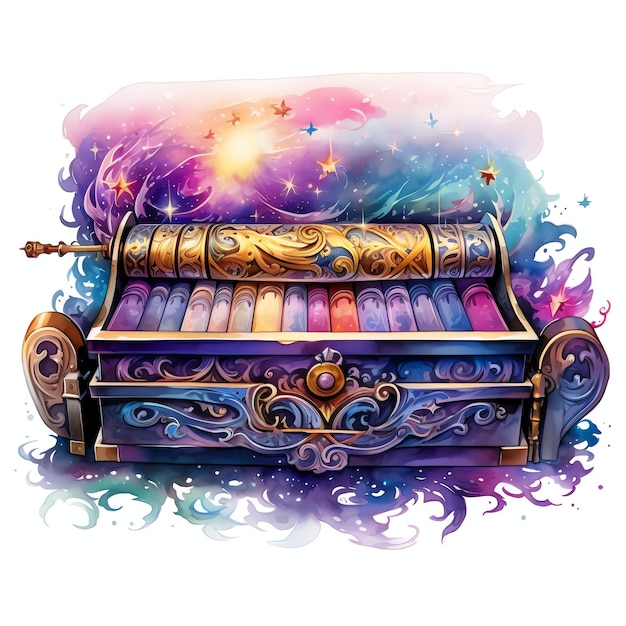The image is a highly intricate artistic design of what appears to be a piano that is uniquely shaped like a dresser or a music box, possibly created digitally. The foreground features an elaborate rectangular structure, with an intricate metalwork design at the front, including a central button flanked by wing-shaped metallic elements. The piano keys themselves are colorful and varied, suggesting a fantasy theme. Inside the top of this object, there are tubes or rolled-up scrolls, including one prominently gilded and colorful scroll. The background is a vibrant blend of flowing colors and patterns, incorporating swirling teals, purples, blues, pinks, and soft yellows, along with star-like elements. These colors and elements weave through and around the central object, enhancing the imaginative and detailed nature of the image. A delicate print resembling a bird is present at the top of the keys, adding to the intricate and fantastical design.